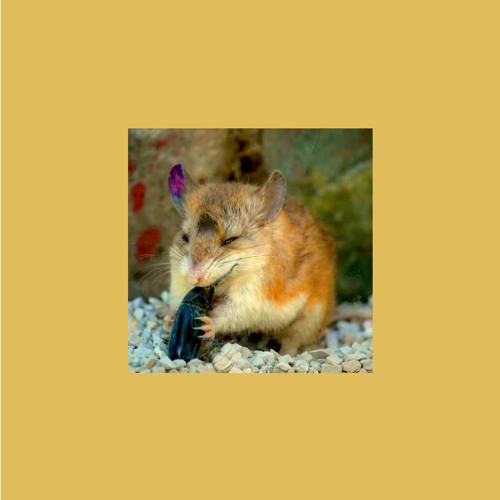In this detailed image, a rodent, possibly a gerbil or hamster, is centrally positioned within a square frame against a brownish-yellow background. The rodent, characterized by a predominantly orange body with white underparts and a brownish-gray head, appears to be eating a black beetle. Its small claws tightly grip the beetle, and there is a noticeable smile-like expression on its face, suggesting enjoyment. The rodent sits on a bed of small, gray pebbles, indicative of an artificial setting such as a terrarium. Surrounding the rodent are blurred red, green, and brown stones, adding to the textured backdrop. Unique colorings in the rodent's ears are visible: one ear displays a normal light pink hue, while the other exhibits vibrant purple and blue tones. The overall composition is framed by an orangish, mustard-colored background.